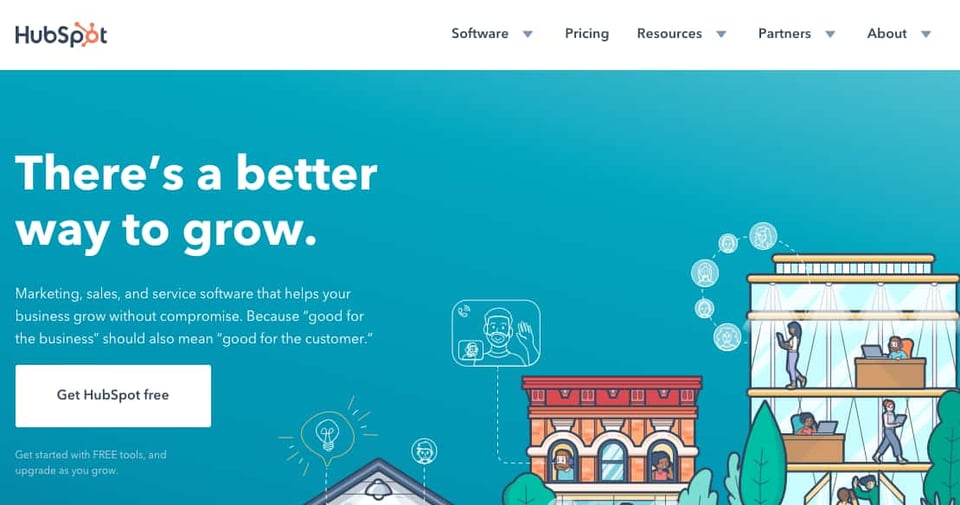The image features a clean white background with "HubSpot" prominently displayed in blue lettering, except for the "O," which is in red and adorned with three small spikes. Below the logo, there are labeled categories: "Software," "Pricing," "Resources," "Partners," and "About," each accompanied by a small blue downward arrow.

The centerpiece of the image is a large blue box containing the text: "There's a better way to grow" in bold white print. The box further elaborates with the message: "Marketing, sales, and service software that helps your business grow without compromise because what is good for the business should also mean good for the customer."

At the bottom of the blue box, a white button with blue text reads "Get HubSpot free." Additional white text below the button states: "Get started with free tools and upgrade as you grow."

Beneath this section, the image showcases three stylized illustrations of buildings, each symbolizing different aspects of business. The first building is topped with two balloons, one featuring a person and the other a lightbulb. The second building is a brick structure with two individuals visible in the upper windows, flanked by small trees. The final building is a multi-story edifice with various people depicted working at desks and moving about the floors. Five small circles emerge from the top floor, extending up to the roof, suggesting growth and upward movement.